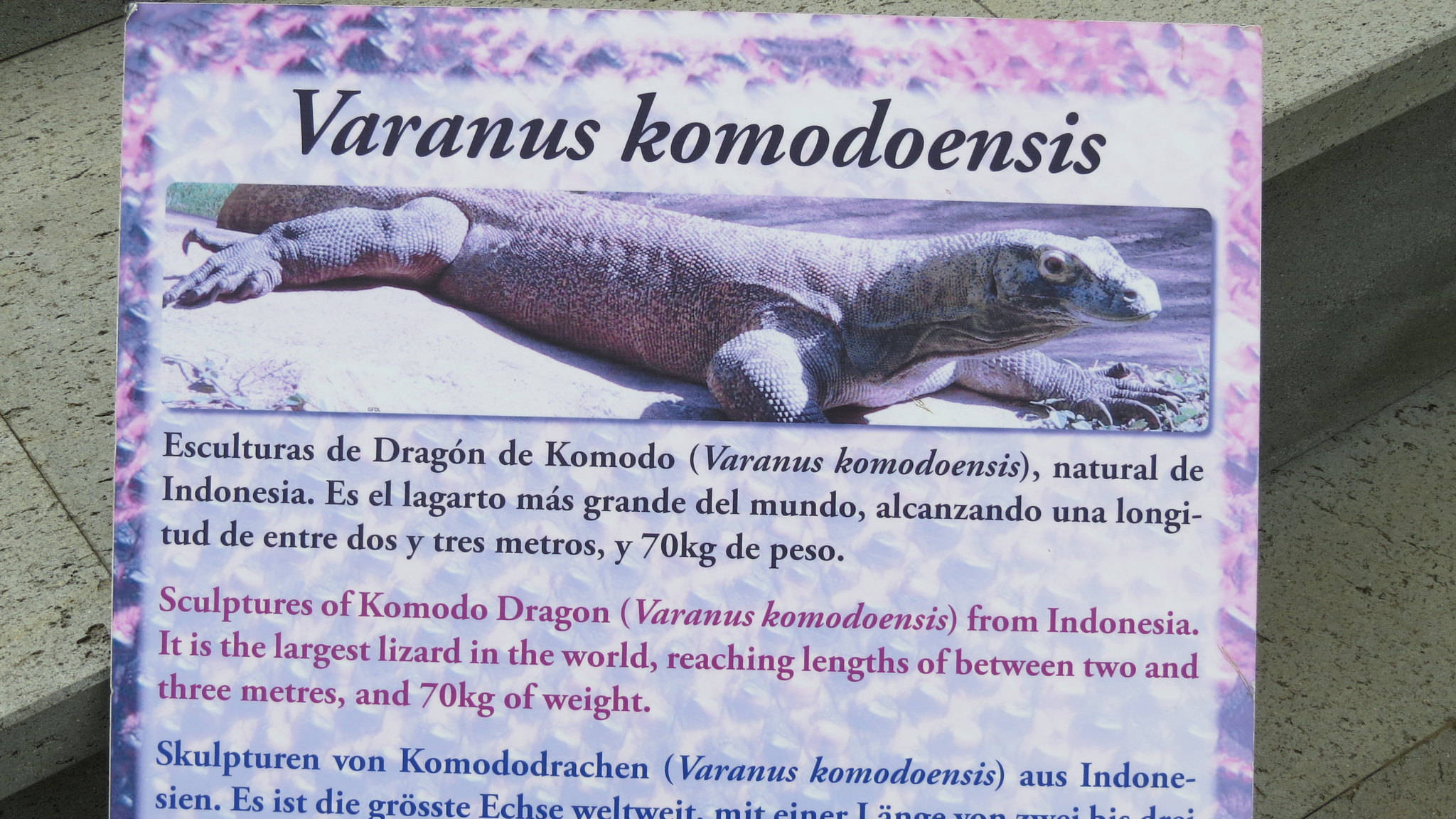The image depicts a detailed informational sign likely found at a zoo, featuring the Komodo dragon. The sign's background emulates the Komodo dragon's skin in shades of purplish-pink, overlaid with a semi-transparent white box containing text and imagery. At the very top, the title reads "Varanus komodoensis," also indicating the common name "Komodo Dragon." Centrally placed within the sign is a photograph of the Komodo dragon in its natural habitat. The text, available in both English and Spanish (in black and pink respectively), and also in German (in blue text), reads: "Sculptures of Komodo Dragon, Varanus komodoensis, from Indonesia. It is the largest lizard in the world, reaching lengths of between 2 and 3 meters and 70 kilograms in weight." This informative sign provides visitors with key details about the Komodo dragon, highlighting its impressive size and origin.